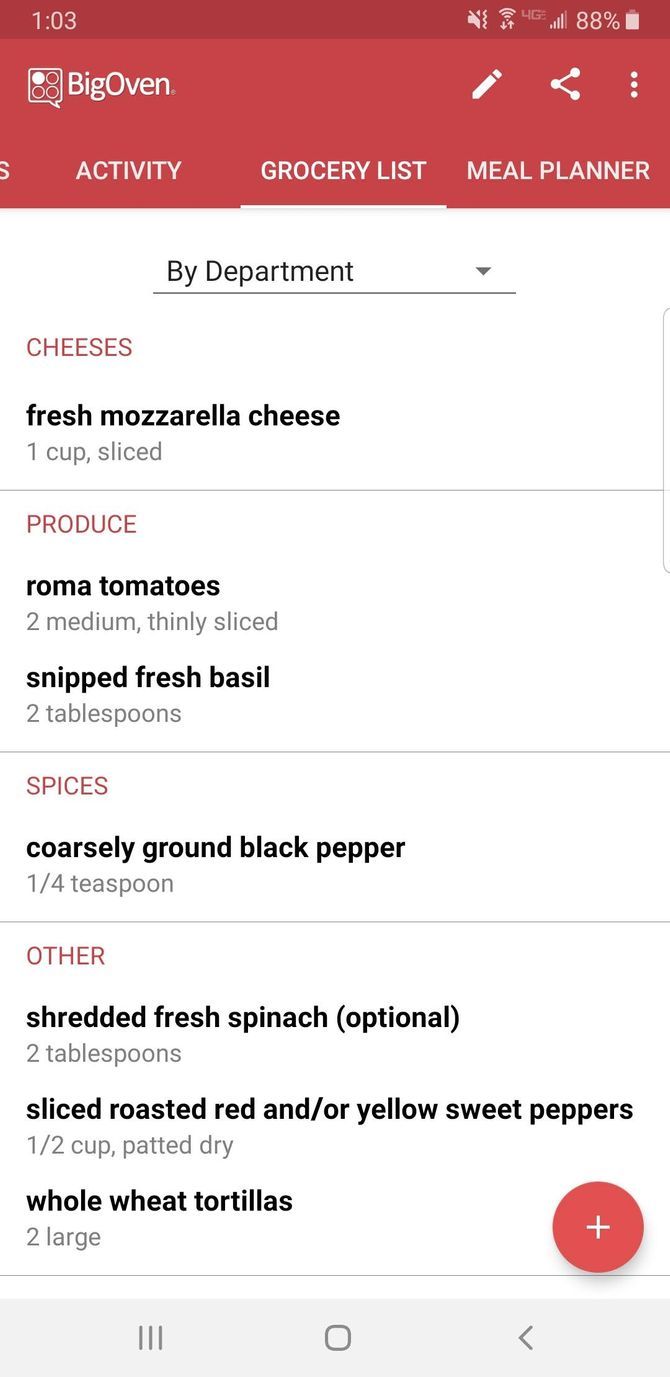The image shows a mobile phone displaying a website. At the very top of the screen is a prominent red bar, which includes icons indicating an 88% battery life, an active internet connection, and the time, which is 1:03.

Below this red bar, the website's interface features the heading "BigOven" accompanied by an icon of a square with white circles inside it. The interface is divided into several sections:

1. **Main Menu**: 
   - *Activity*
   - *Grocery List*
   - *Meal Planner*

2. **Grocery List Items by Department**:
   - **Cheese**: "Fresh Mozzarella Cheese, one cup, sliced"
   - **Produce**: "Roma Tomatoes, two medium, thinly sliced" and "Snipped Fresh Basil, two tablespoons"

3. **Additional Ingredients**:
   - **Spices**: "Coarsely Ground Black Pepper, a quarter of a teaspoon"
   - **Other**: 
     - "Shredded Fresh Spinach (optional), two tablespoons"
     - "Sliced Roasted Red and/or Yellow Sweet Peppers, half a cup, patted dry"
     - "Whole Wheat Tortillas, two large"

Each item in the list is displayed neatly, and adjacent to some ingredients is a red circle with a white plus sign, likely for easily adding items to the list.

The website's overall design features a clean, white background, making the red bar and other elements stand out for better readability. The bottom of the screen displays various icons, indicating additional functionalities available within the app.